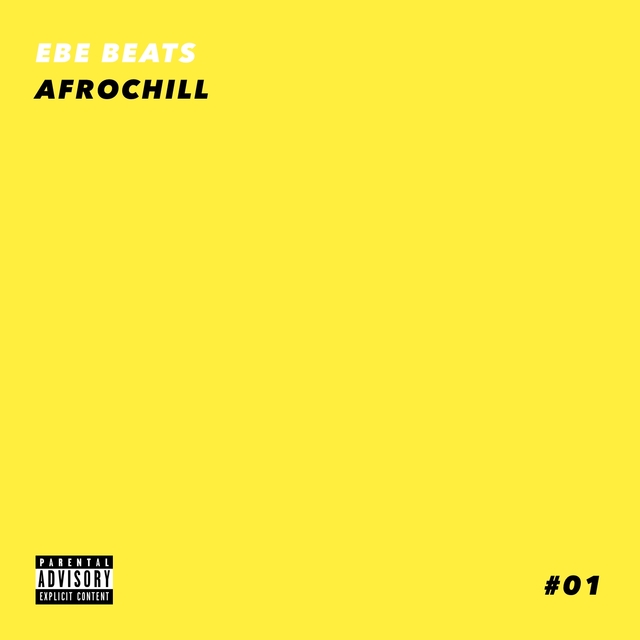The image is a vibrant, bright yellow square that appears to be a cover for a CD or a music album. In the upper left-hand corner, it features the text "EBE BEATS" in prominent white capital letters. Directly below this in black capital letters is the word "AFROCHILL." The bottom left-hand corner displays a black and white Parental Advisory Explicit Content box, commonly seen on albums containing explicit material. Additionally, in the bottom right-hand corner, there is a hashtag (#) followed by the number "01" in black font, possibly indicating the debut release from this artist or group. The overall design is minimalist yet striking, dominated by the single bright yellow color with text elements providing essential information.